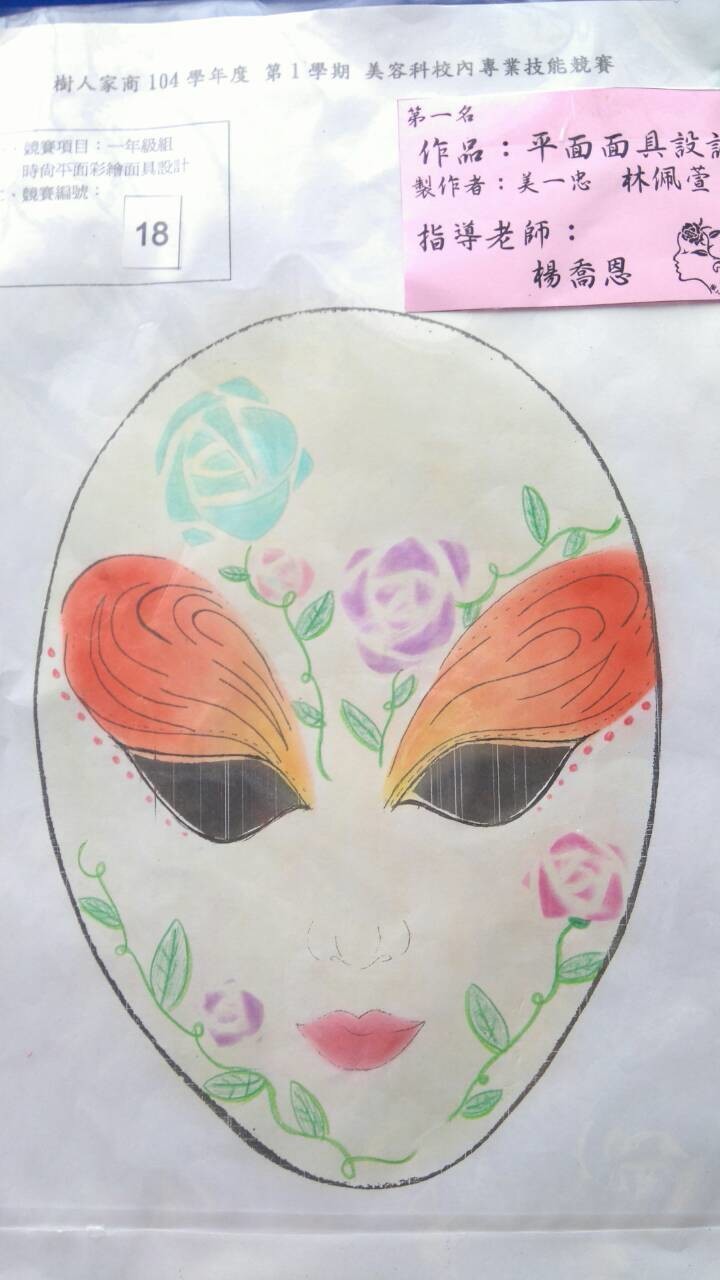The photograph captures a detailed illustration on what appears to be wrinkled silk, characterized by visible vertical fibers and a predominantly white background. At the top of the image, small Chinese characters are inscribed above a piece of pink paper containing handwritten Chinese text and a small doodle on the right side. The central focus is the depiction of a face shaped like an upside-down egg, suggesting it might be a mask. This face is adorned with large black almond-shaped eyes, framed by orange butterfly wing-like eyelids with intricate black lines. The bridge of the nose is subtly shaded in light gray, while the tip and nostrils are more defined. Embellished with blue and purple roses, alongside pink and red blossoms with tendrils, these floral designs stretch across the forehead and cheeks, rendered in a stencil-like style for the petals and leaves. The cheeks are lightly colored pink, and a tendril-like plant frames the face from the upper cheeks to the chin. The image also includes a rectangular outline featuring a smaller square with the number 18 and additional Chinese writing, giving the appearance of a label.